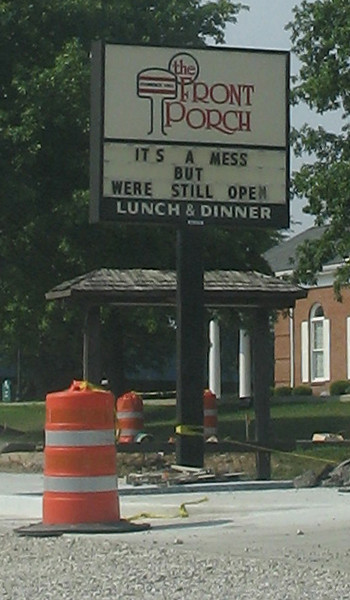The exterior photograph captures the entrance to a restaurant amid a construction zone. Central to the image is a tall, rectangular sign with a white base outlined in a black border. At the top, in elegant red lettering, it reads "The Front Porch," with the word "The" circled within a black border. Towards the bottom left, the sign morphs into a tall pole, capped by a hamburger-shaped illustration. Beneath this, a black divider separates the upper portion from the message below, which states in black letters, "It's a mess but we're still open." Further down, white capital letters on a dark backdrop announce "LUNCH AND DINNER."

The black rectangular pole of the sign is encircled by caution tape at its base. Littered around the site are construction cones—large, cylindrical, and orange with two white stripes. One prominent cone in the foreground also has caution tape protruding from its top. Surrounding the sign is a debris-strewn road, indicative of ongoing construction. In the background, a brick building features a black slate roof, white trim, and an arch-shaped window with white shutters. Trees and a hazy blue sky frame the scene, adding to the overall atmosphere of renovation and resilience.